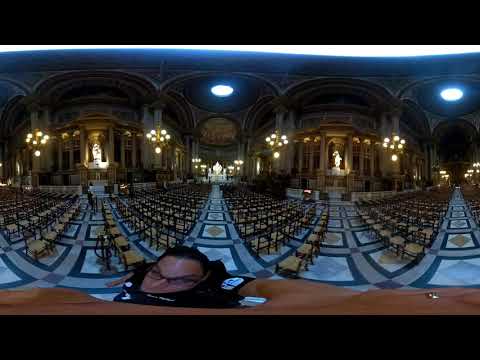A young man, likely using a fisheye lens or a panoramic image filter, captures a surreal selfie inside a grand, dimly-lit interior that resembles a cathedral or church. The distortion from the lens warps his face and the surrounding architecture. He stands in the middle of an aisle lined with numerous unoccupied seats instead of traditional pews. The floor beneath him features intricately designed tiles forming bordered squares with white centers and central diamonds. The setting is adorned with multiple arches and pillars, with a well-lit altar area at the aisle's end, where a priest would typically stand, suggesting a Catholic affiliation. Behind the altar, a statue surrounded by pillars is faintly visible. The young man, dressed in a black shirt with a visible patch on his left arm, holds his smartphone with his left hand, wearing dark glasses. The image is slightly cropped with a black border at the bottom, emphasizing the dramatic and almost ethereal atmosphere of the scene.